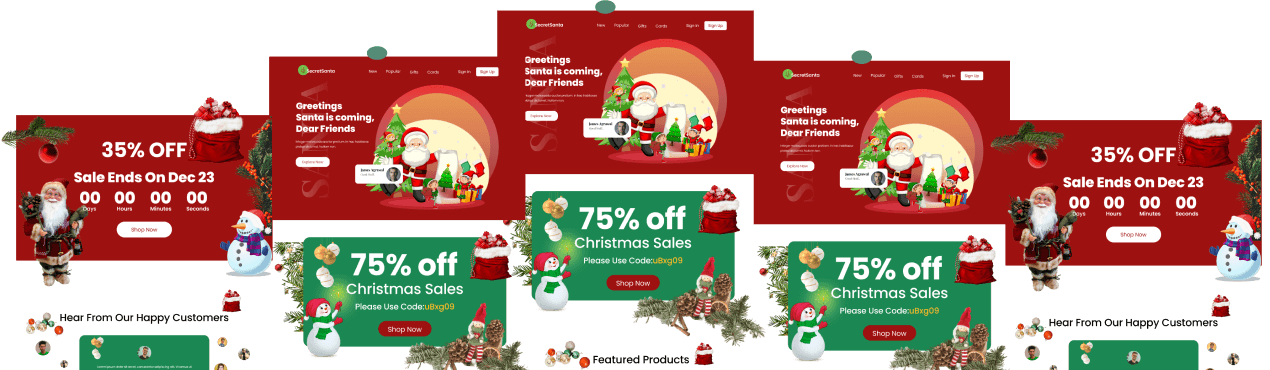The image showcases a composite view of five different website screenshots, each prominently displaying a holiday-themed design. The overall layout resembles a vertical pyramid, with the widest part at the bottom composed of three central screenshots, and two additional ones placed above. Each website features a red background reminiscent of Christmas colors, giving a cohesive festive look.

At the top of each screenshot, there is a navigation menu, typical of website layouts, followed by various banners and promotional elements descending downwards. The three central screenshots share an identical banner showing Santa Claus standing next to an animated Christmas tree positioned on the left side of the frame.

The two outer screenshots, located on the left and right, contain white text over the red background, announcing a "35% off" sale that ends on December 22nd. Each section of the screenshots displays a timer, which has counted down to zero, across four different segments, indicating the end of the promotional period. Despite the small size of the images, the festive and promotional themes are consistent throughout, underscoring a cohesive holiday marketing campaign.